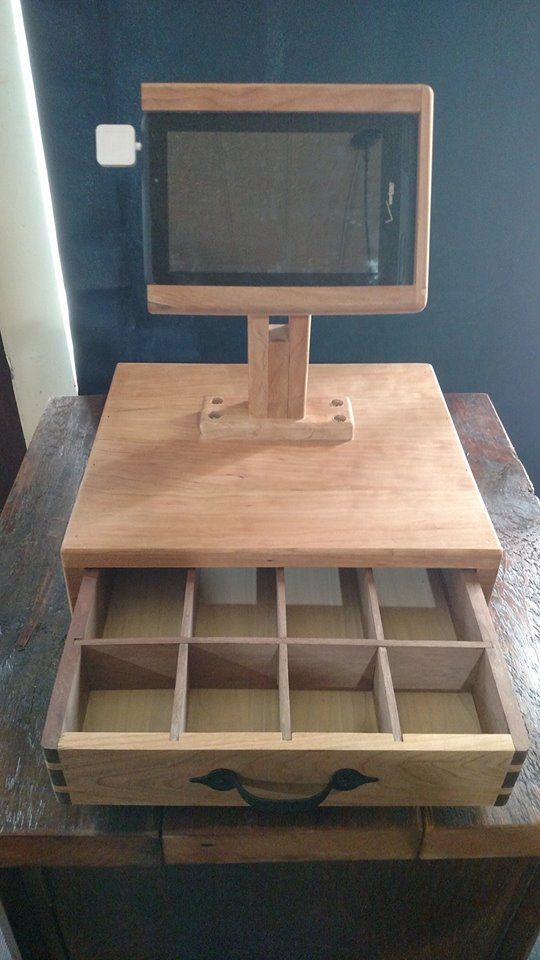This indoor photograph features a meticulously handmade wooden cash register model set atop a dark brown wooden table. The cash register itself is a light brown, perhaps made from unfinished maple or pine, showcasing various shades of natural wood. The central component is a large square wooden box with a partially opened front drawer featuring a black handle. Inside this drawer are eight neatly arranged compartments, possibly for organizing money.

Above the drawer, a sturdy wooden stand is intricately designed to hold a black, plastic-frame tablet, which appears to be an iPad with its screen turned off. To the left of the tablet, a small white plastic square, likely a credit card reader, is affixed, adding to the authentic feel of the setup. The background includes a black curtain with a glimpse of a white wall and a white post in the upper left corner, with light coming from the right, casting a slight shadow to the left. The detailed craftsmanship and functional design elements suggest a unique blend of artistry and practicality, resembling a modern-day cash register.